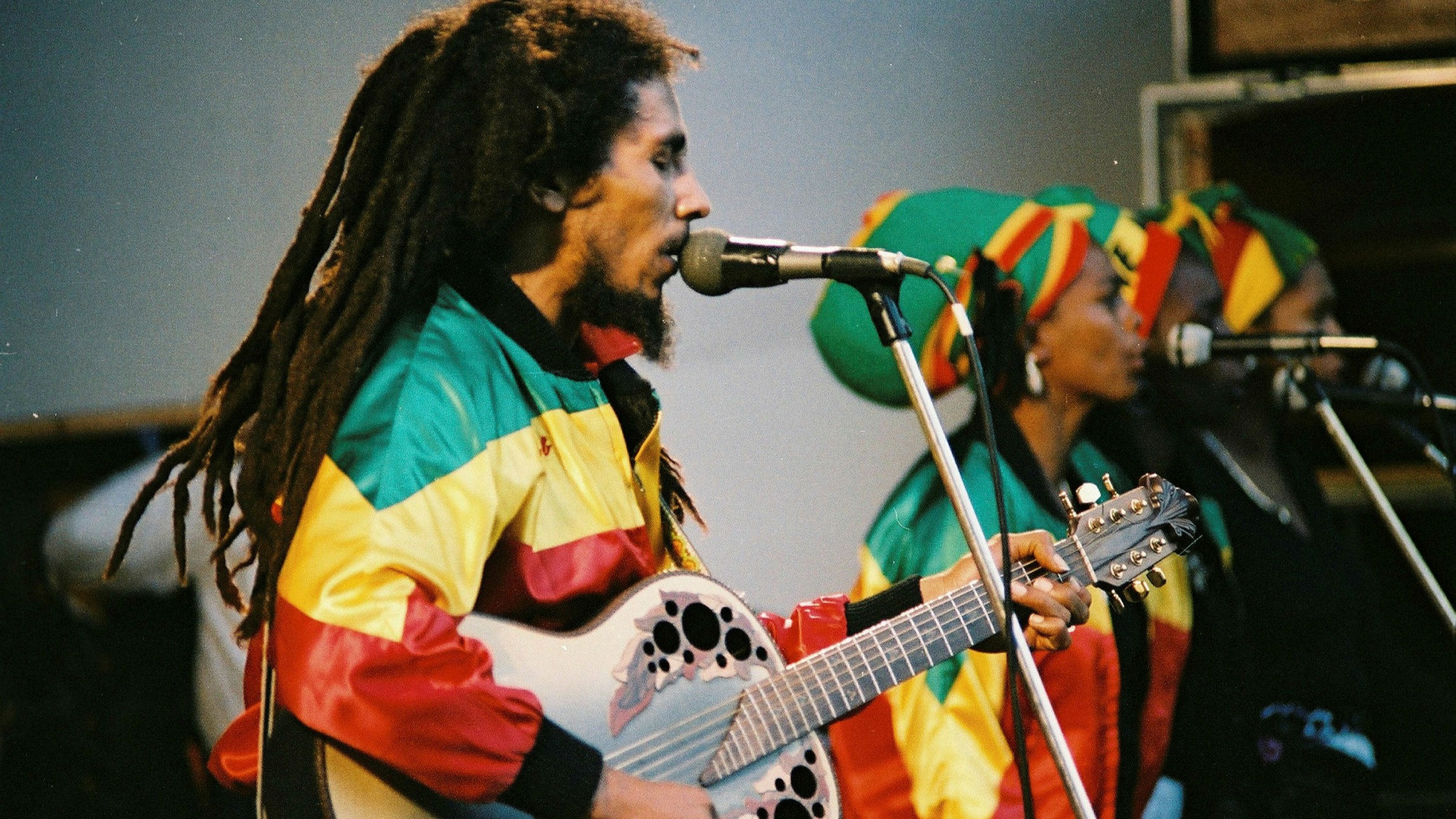This image captures an electrifying performance by reggae legend Bob Marley. Centered on stage, Marley is depicted with his long, dark brown dreadlocks cascading down to the middle of his back and a scraggly black beard adorning his face. Dressed in a vibrant green, yellow, and red jacket, reflecting the colors of Jamaica, he passionately sings into a gray microphone mounted on a black stand, while cradling a white electric guitar with a light gray to blue neck and gold-plated tuners.

Flanking Marley, on the right side and rear of the stage, are three female backup singers. They too are dressed in matching green, yellow, and red jackets, with coordinated headscarves that pull back their hair in a traditional style. Some of the women are also wearing earrings. Each woman stands before a microphone, adding harmonies to the performance.

The backdrop features a modest setup with black, brown, and white amplifiers or speakers framed in silver, contributing to the intimate yet dynamic atmosphere of this vintage scene, likely from the 1970s. The photo, though showing some grain, captures the spirited essence of Bob Marley's enduring legacy in reggae music.